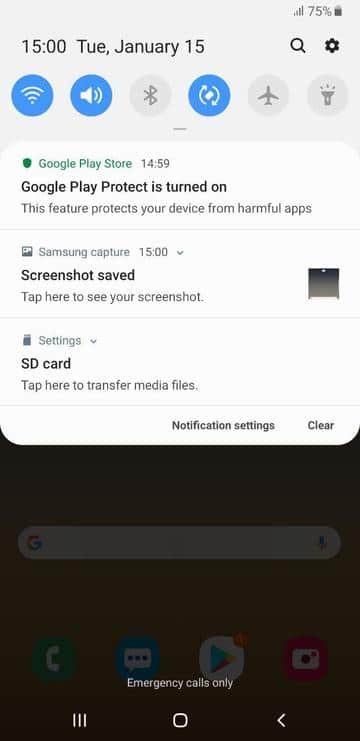A screenshot displaying a blurred Google Play Store page is centered on the image. At the very top, the screen indicates the time as 15:00 hours on Tuesday, January 15th, shown on the left side. On the right, an hourglass icon and a battery indicator displaying 75% are visible. Just below, various icons, including sound controls, airplane mode, and three additional symbols, are depicted.

Underneath this row of icons, a green notification indicates an action on the Google Play Store at 14:59. Following this, a message from Google Play Protect reveals that the feature is activated, ensuring the device is safeguarded from harmful apps. Further down, another blurred notification from Samsung Capture, timestamped at 15:00 hours, states "Screenshot saved" and prompts the user to tap and view it.

The next notification suggests accessing settings for an SD card, guiding the user to tap for media file transfer options. On the right side along the middle of the screen, clickable options for notification settings and clearing notifications are noticeable.

The bottom section of the screen is enveloped in a murky dark brown color, displaying a blurred Google search bar line. Faded logos appear beneath this bar. At the lowest part of the screen, text indicating "Emergency calls only" is centrally positioned.